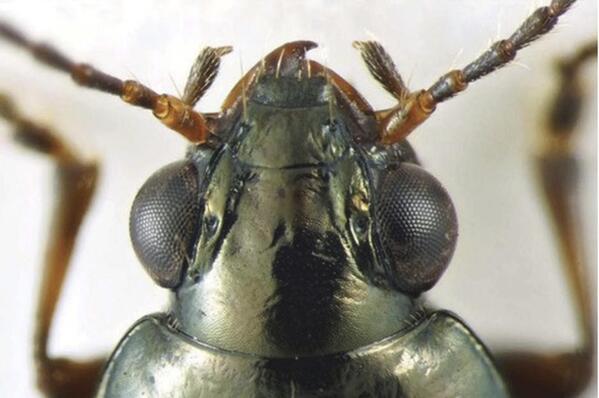The extremely close-up photograph captures the intricate details of a beetle's head and part of its body, with a focus on its vivid, metallic silver-green carapace. Two large, half-spherical eyes, dappled with tiny black dots, dominate either side of the head, nearly pixelated due to the high magnification. Extending from in front of these eyes are two segmented antennas, striped in shades of brown and black, which stretch out of the frame. Although the front legs, colored in brown and tan hues, are visible, they are slightly blurred, emphasizing the depth of field in the image. The beetle’s mandibles extend from its mouth, set against a flat white surface, adding to the striking and reflective qualities of its appearance. This highly detailed and zoomed-in perspective offers a fascinating glimpse into the micro world of this beetle, highlighting its textures and colors vividly.